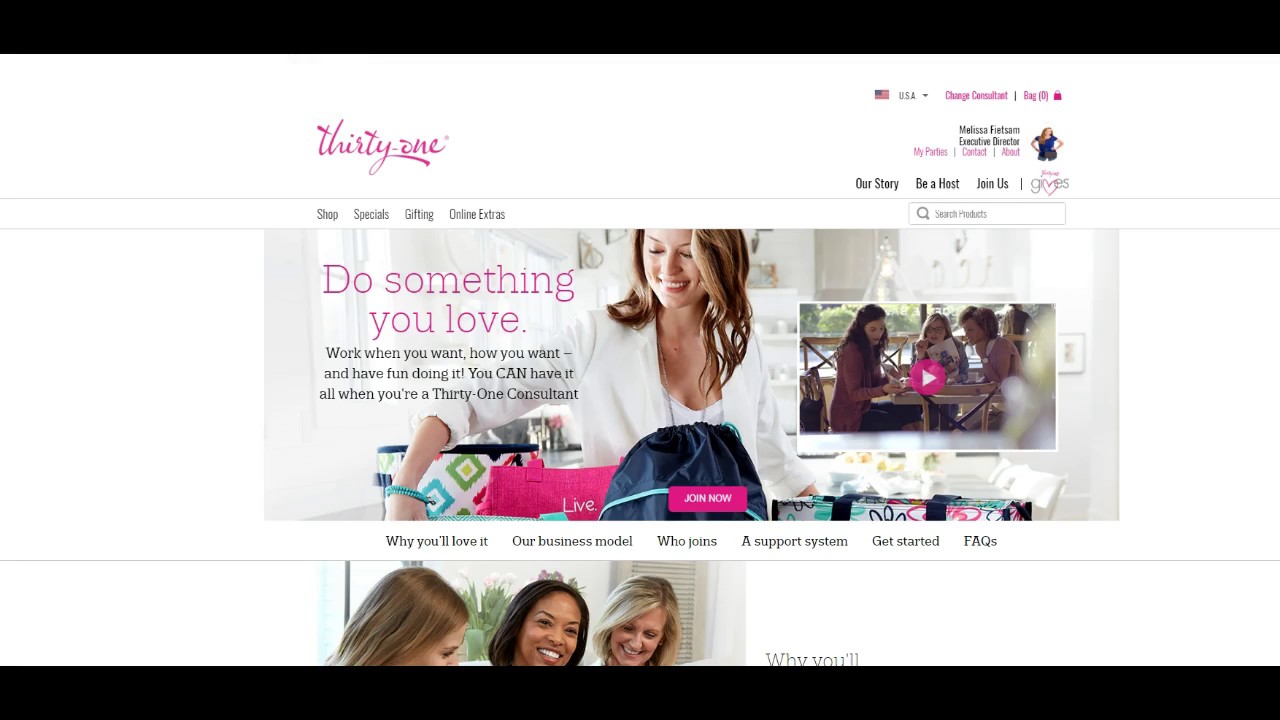This is a detailed caption describing an online storefront webpage:

---

On the left side of the webpage, there's a section titled "31" positioned somewhat in the middle. Beneath this title, the text reads: "Shop Specials," "Gifting," "Online Extras." Moving to the right, you see a drop-down menu labeled "USA" followed by "Change Consultant," "Bag (0)," and the name "Melissa Feitzman, Executive Director." Melissa's last name is spelled F-I-E-T-S-A-M. The navigation bar continues with options: "My Party," "Contact," "About Our Story," "Be a Host," "Join Us," and a feature named "Gives" (though its purpose is unclear).

Below this menu, a search bar allows users to input their queries, accompanied by a search icon. This bar is aligned with the main navigation on the other side of the page. 

The main visual consists of a photograph depicting a woman who appears to be shopping. To the right of her image, the text reads, "Do something you love" in a pinkish-red color, followed by the text "Work when you want, how you want, and have fun doing it" in black. An additional message declares, "You CAN have it all when you are a 31 consultant," emphasizing the word "CAN" in capital letters.

Adjacent to this text, there's a small circular video play button in pink, featuring a white right arrow. Below this is another set of navigational links: "Why You'll Love It," "Our Business Model," "Who Joins," "Support System," "Get Started," and "FAQs."

The layout suggests that more content follows further down the page.